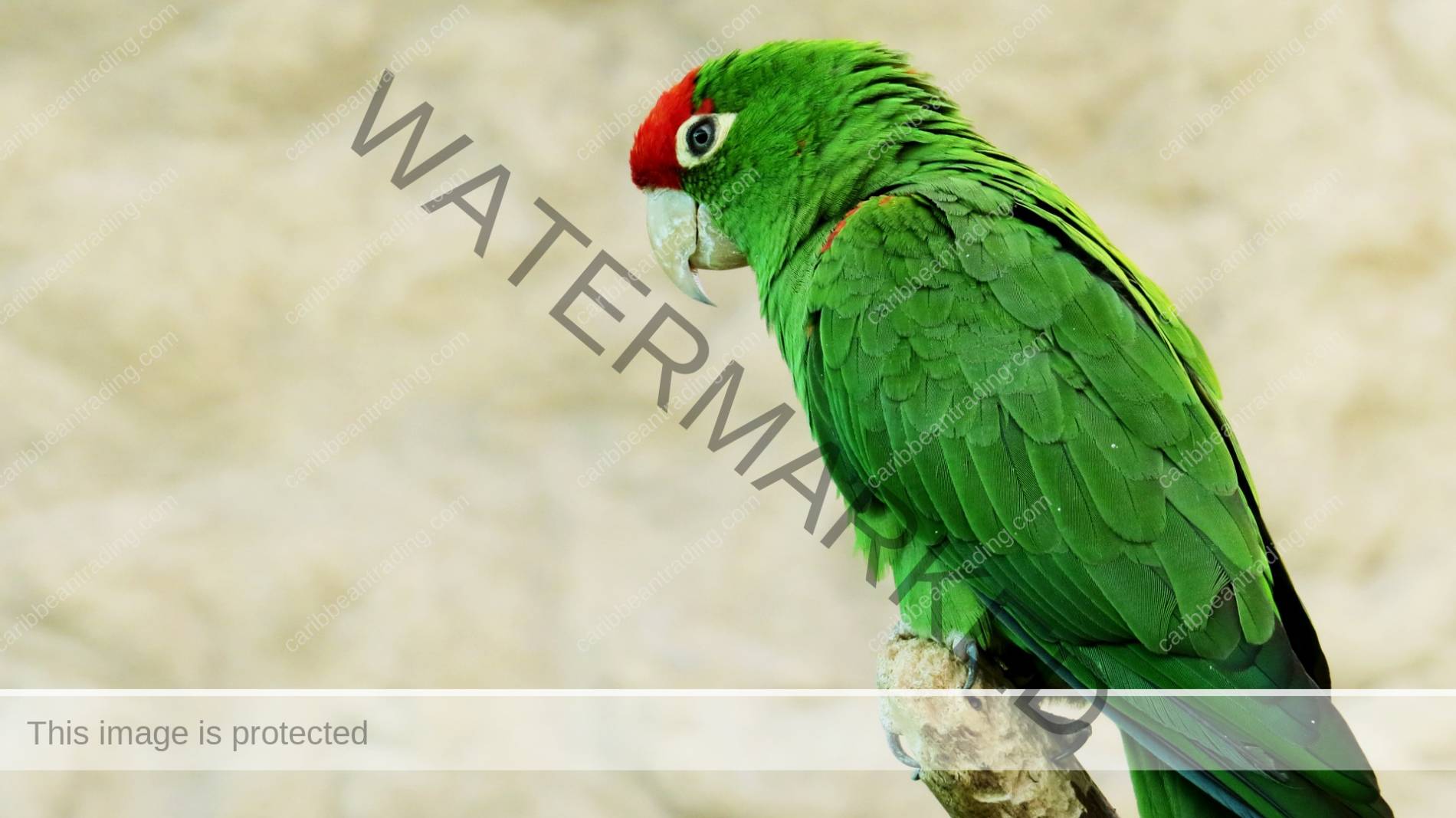This professional full-color photograph displays a vibrant green parrot perched on a small nub of wood, captured using natural light. The image is horizontally rectangular and taken outdoors, though the subdued background—a blend of whites, grays, and browns—leaves its exact location ambiguous. The parrot, facing left, reveals nearly its entire body, prominently displaying its predominantly green plumage with a vivid red forehead and eye area, along with subtle highlights of lime green throughout its feathers. The beak is a light tan color, and just above the wing shoulder is a hint of red. The eye has a distinctive white ring around it. Part of the tail, slightly blurred in the background, exhibits faint traces of blue and black. The photograph is watermarked twice: a large gray "watermarked" text diagonally across the middle, and another watermark from "Caribbean Trading.com." Moreover, a tan banner extending from the bottom left to the bottom right corner states, "This image is protected."